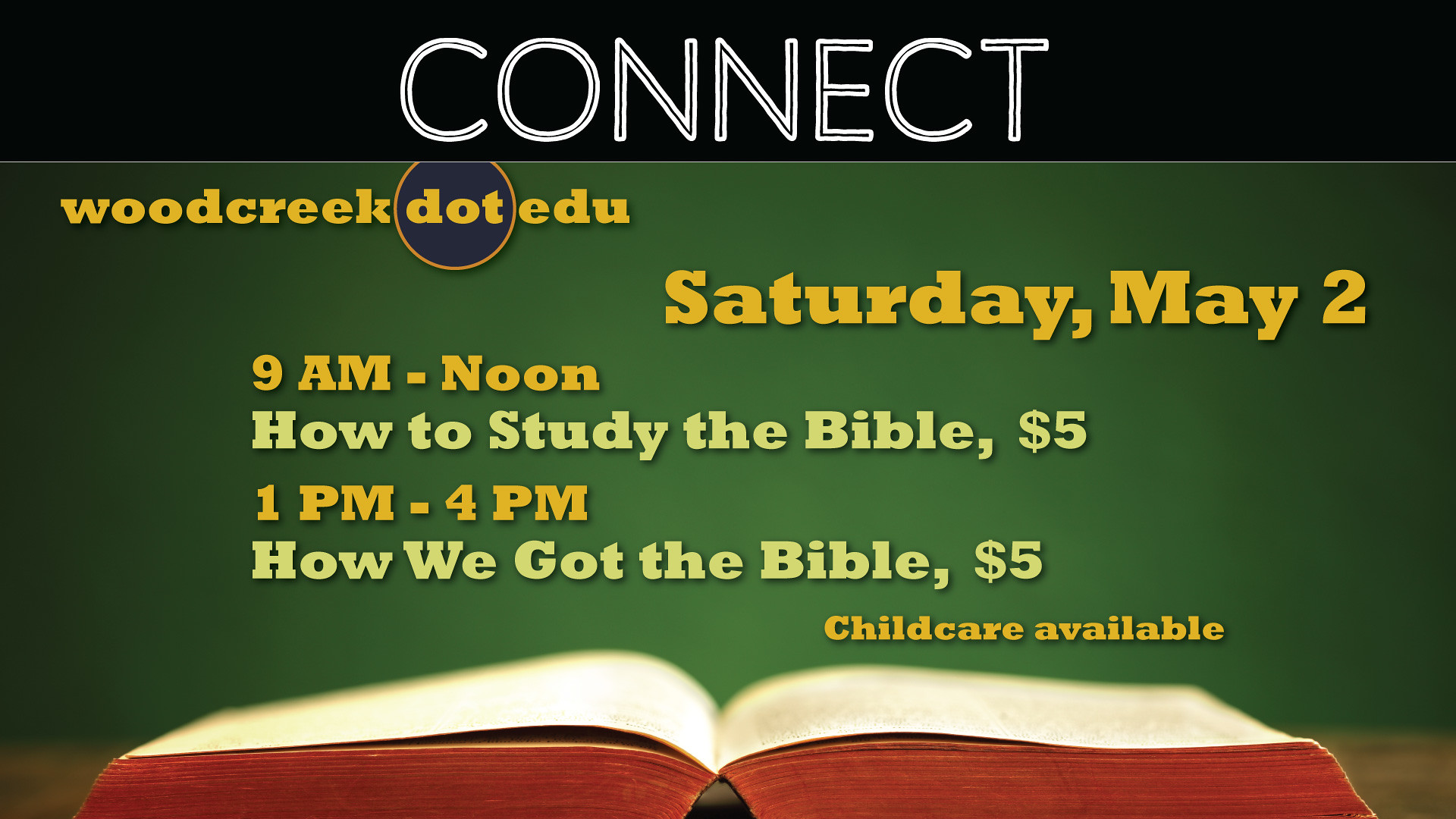The image is a horizontal flyer with a predominantly green background and uses yellow and green text for emphasis. At the top, there is a black banner with the word "Connect" prominently displayed in white text. Below this banner, a URL "woodcreek.edu" is printed in yellow text, framed by a blue circle with a yellow outer ring. The event details follow: "Saturday, May 2nd," and "9 a.m. to noon," both in yellow. The next line in green text reads "How to Study the Bible, $5." Further down, another time slot, "1 p.m. to 4 p.m.," is listed in yellow, followed by the green text "How We Got the Bible, $5." Below these details, "Childcare available" is written in yellow. An open Bible, with its pages appearing brightly colored, is illustrated at the bottom of the flyer.